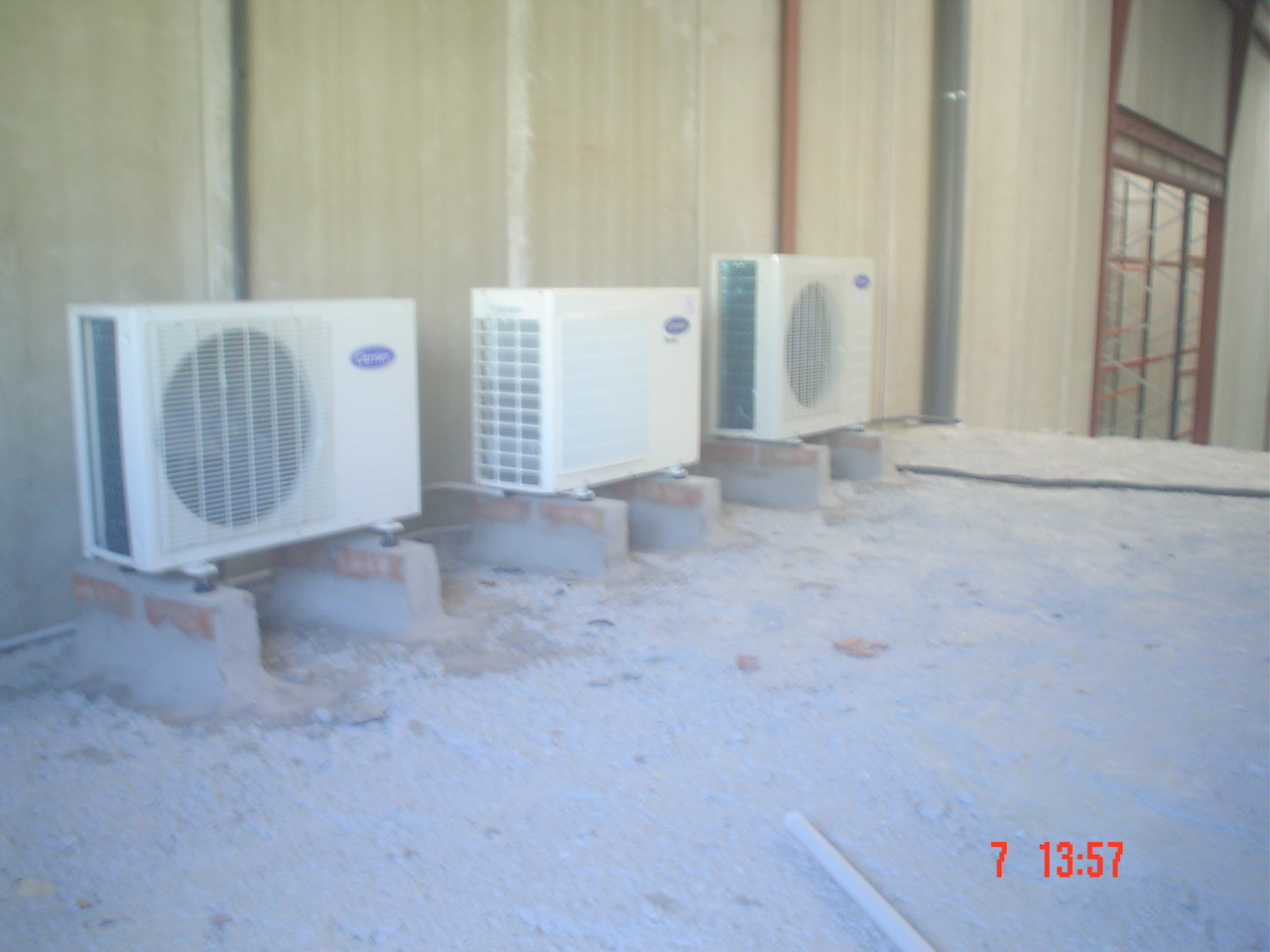This image appears to be taken from an old digital camera and captures a construction site featuring the exterior of a building with part of its structure being higher and another part lower, suggesting a tiered roof design. Central to the image are three off-white mini-split air conditioning units, each elevated on cinder blocks and cement. Two of these units feature large round grilles for air exchange, while the middle one is distinguished by a square grille. All three units bear a brand logo in purple and white coloring. These units are aligned in a row against a tan concrete wall, which also has visible water and piping lines extending from the mini-splits. The ground below is covered in dusty concrete and dirt, characteristic of an active construction zone. Notable in the background, through what appears to be a large glass door with a brownish trim, there is a structure resembling scaffolding. In the bottom right corner of the image, a timestamp in red reads "7, 13:57," possibly indicating the 13th minute and 57th second of recording.